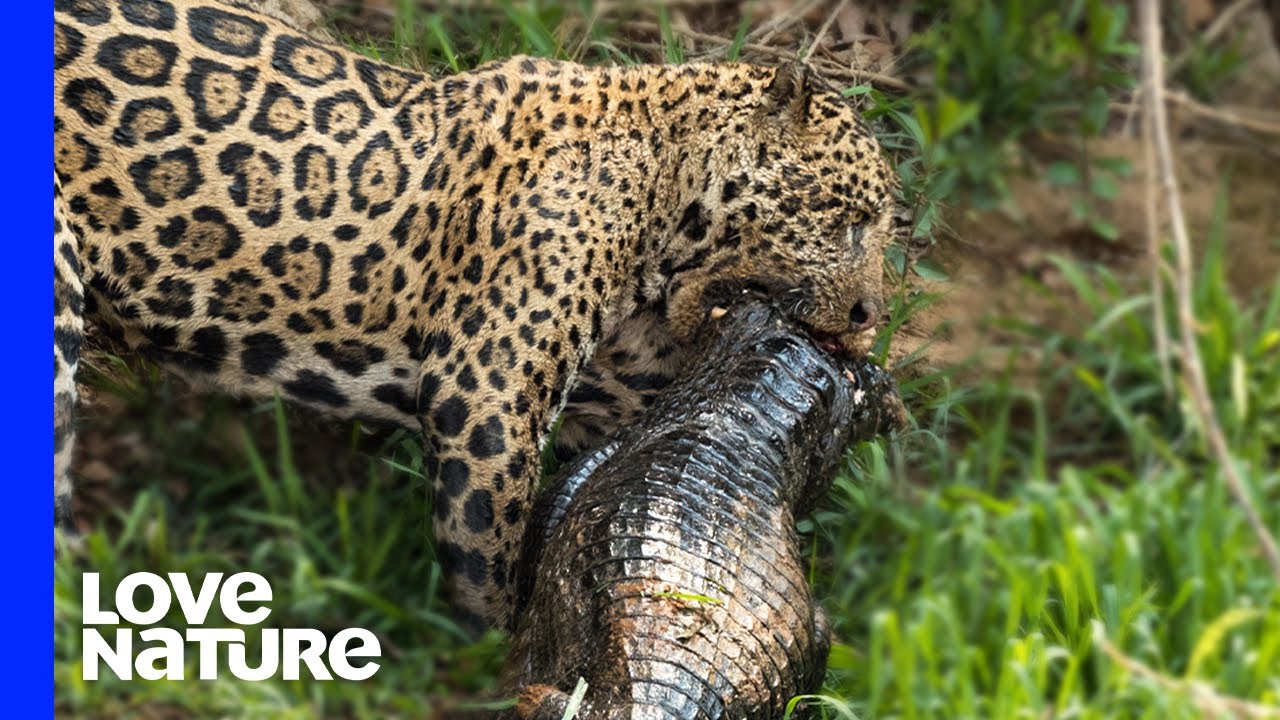In this captivating image, a side profile of a majestic leopard is depicted. The leopard's powerful jaws are clamped around the neck of an alligator, its face and fur visibly wet, likely from the struggle. The setting is a lush, wild landscape with tall, golden grasses surrounding the two creatures, and a fallen tree trunk can be seen in the distance amidst the greenery. The leopard's tan coat, patterned with distinctive black spots, contrasts with its black nose and short, erect ears. Its striking golden eyes gaze intently ahead. In the lower left-hand corner, the words “Love Nature” are inscribed in white letters, emphasizing the raw and untamed beauty of the natural scene.